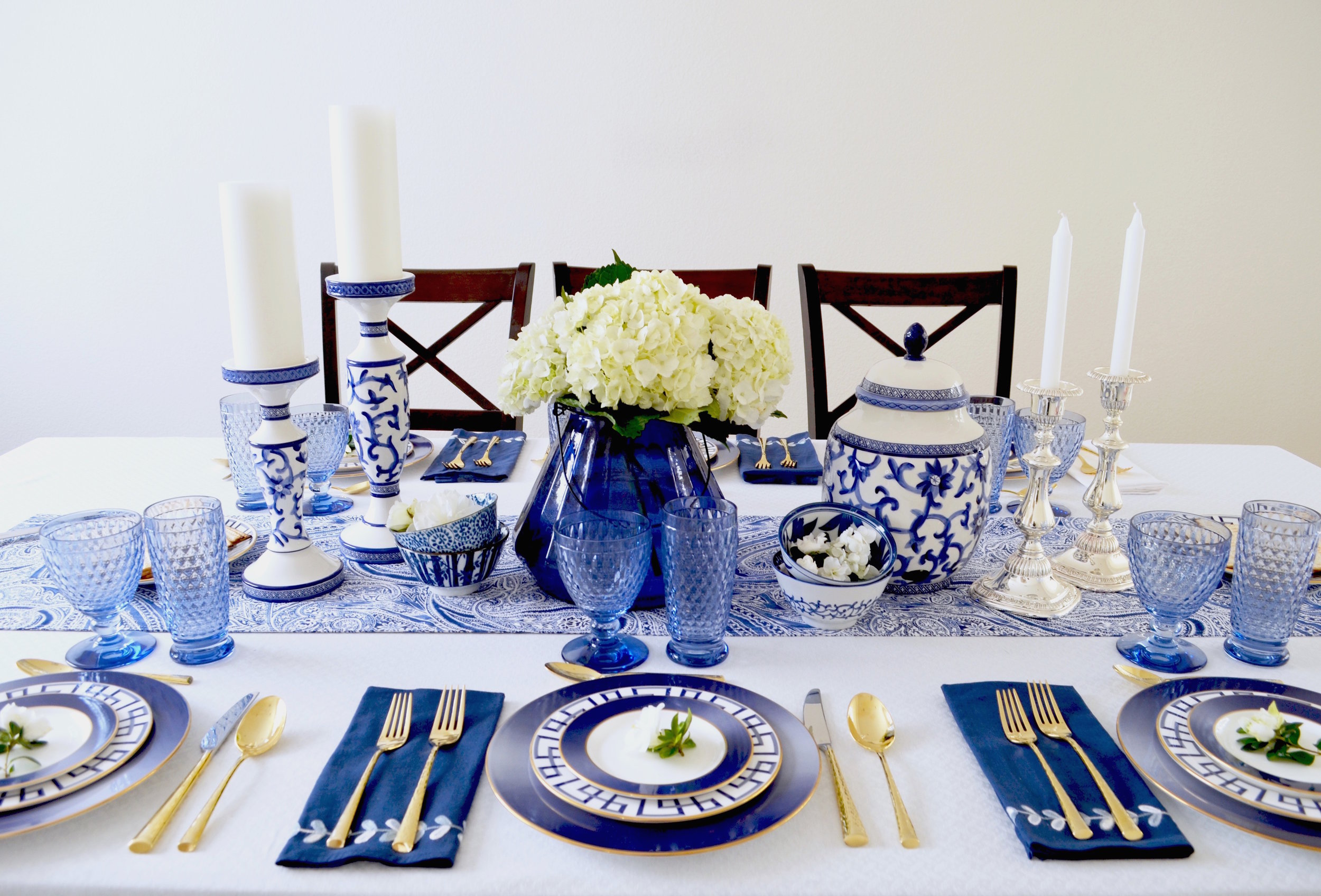This detailed photo captures a meticulously staged indoor dining scene, focusing on a blue-themed table setting against an off-white wall. The square image showcases a rectangular dining table covered with a pristine white tablecloth, flanked by three wooden chairs on the opposite side. Centrally, a blue runner with intricate patterns extends down the middle.

On the table, each of the six settings features a blue ceramic plate adorned with white floral decorations, complemented by blue napkins with white embellishments. In front of each plate, there are two blue glass cups, and atop the plates sits gold-colored cutlery, including knives, spoons, and two forks, placed underneath the napkins.

The centerpiece is a striking blue vase brimming with a bouquet of white flowers, providing a refreshing contrast. This is flanked by four candle holders: two substantial blue-and-white patterned holders with white candles, and two smaller silver holders, also with white candles.